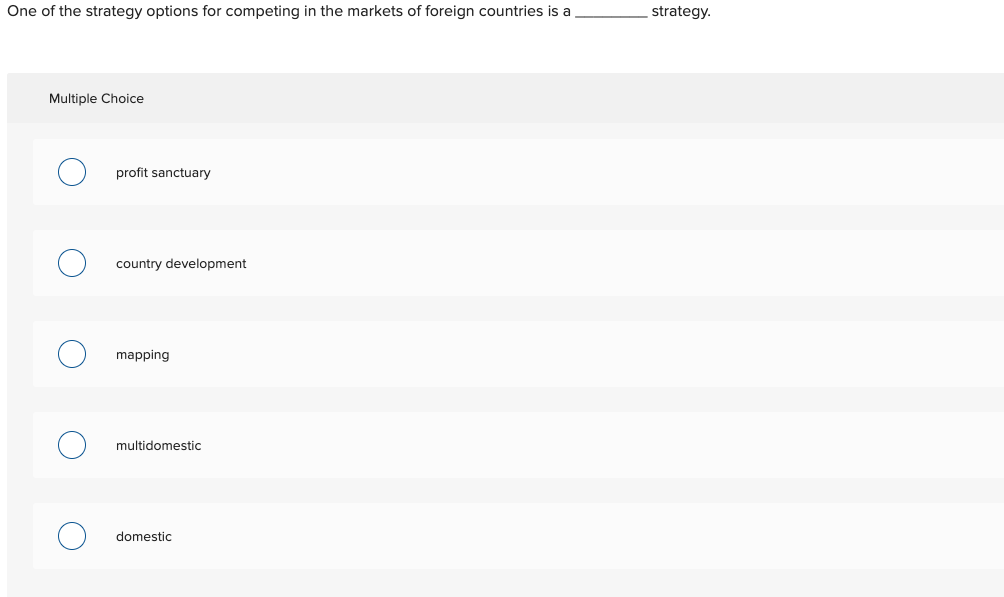At the top of the image, a question in black text reads, "One of the strategy options for competing in the market of foreign countries is __________ strategy." Beneath the question, there are multiple choice options listed as follows: profit, sanctuary, country development, mapping, multi-domestic, and domestic. Each option is accompanied by a blue circle with a white center, all outlined in a faint light blue line. The options are placed on a gray background with a white bar underneath each option. None of the circles have been selected. The overall color scheme of the image features black, blue, gray, and white. Notably, the phrase "multiple choice" is capitalized, while the individual answer choices remain in lowercase. The image appears to be a question from a larger document or quiz, with no additional context provided.